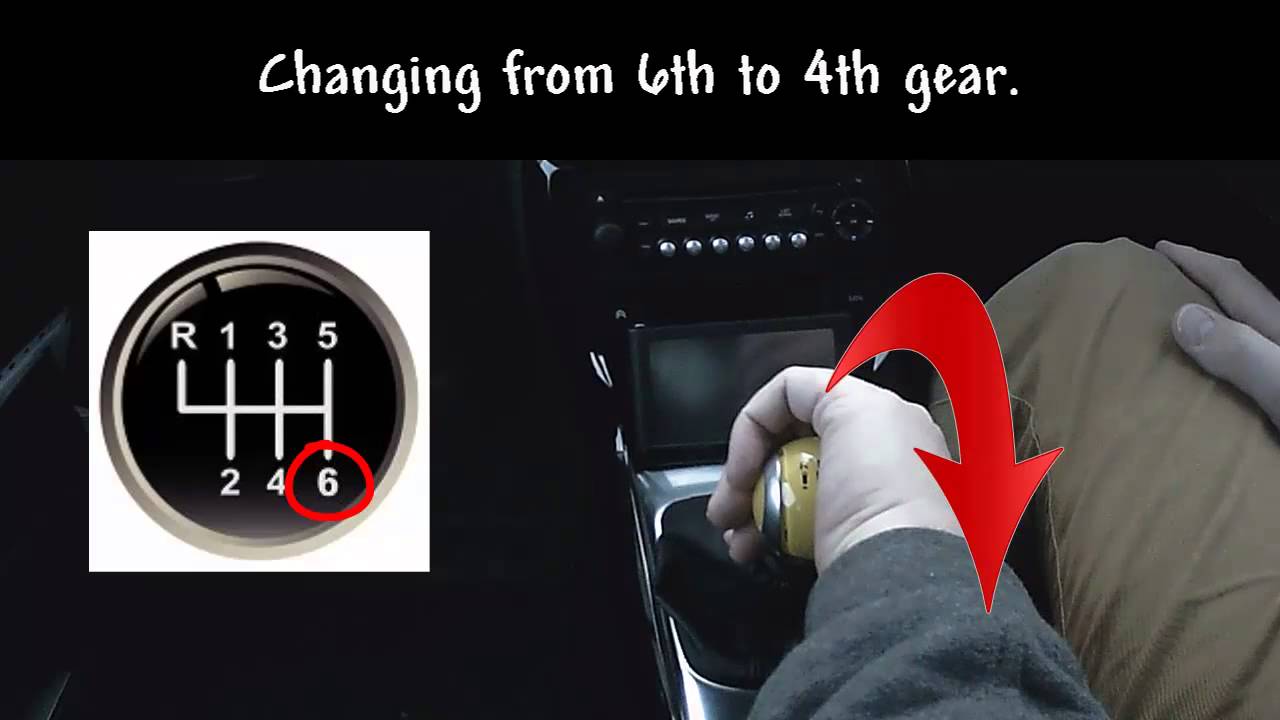The image is a horizontal rectangular illustration titled "Changing from Sixth to Fourth Gear," prominently displayed in white text against a black background at the top. The scene is set inside a car, focusing on the center console area. In the middle of the image, a hand grips a gear shift with a distinctive white or yellow and silver ball atop it, marked with a red directional arrow indicating to pull the shifter backward. Below the text and to the left, there's a detailed diagram showing the gear positions in this particular shift pattern: 'R', '1', '3', and '5' are arrayed across the top row while '2', '4', and '6' run directly below them, with '6' circled in red. The background suggests dim lighting inside the vehicle, with the console and radio buttons visible in front of the shift. The driver appears to be seated on the right side of the car, using the left hand to maneuver the gear shift, which can be confusing due to orientation. The image aims to instruct on how to shift from sixth gear to fourth gear in a manual transmission vehicle.